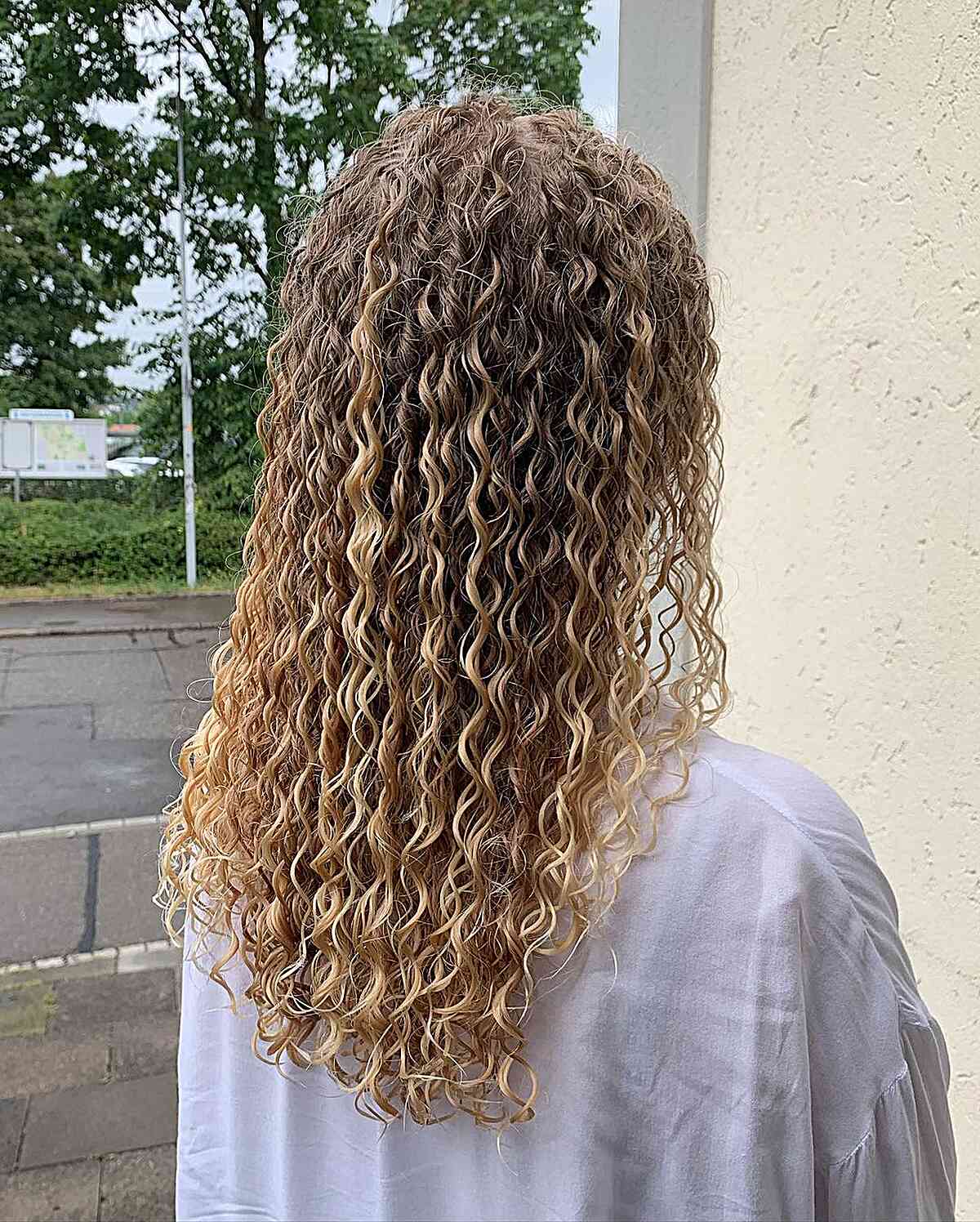In the image, there is the back of a person's head centered, showcasing wavy, brown hair that cascades down to their upper back, possibly reaching the midpoint of their shoulder blades. They are dressed in a white, somewhat translucent top, through which faint bra straps are visible, indicating the person is likely female. This individual is facing an off-white or tannish stucco wall on the right side of the image, suggesting they are standing or sitting upright, although the photo cuts off at their chest. On the left side of the image, a vibrant outdoor scene unfolds featuring a large tree with green leaves, a grassy area, and a street that appears slightly damp, hinting at recent rain. Alongside the road, which has a greenish hue, there's a sidewalk with a pole and a signboard. The blue sky above solidifies that this photo was taken during the daytime.